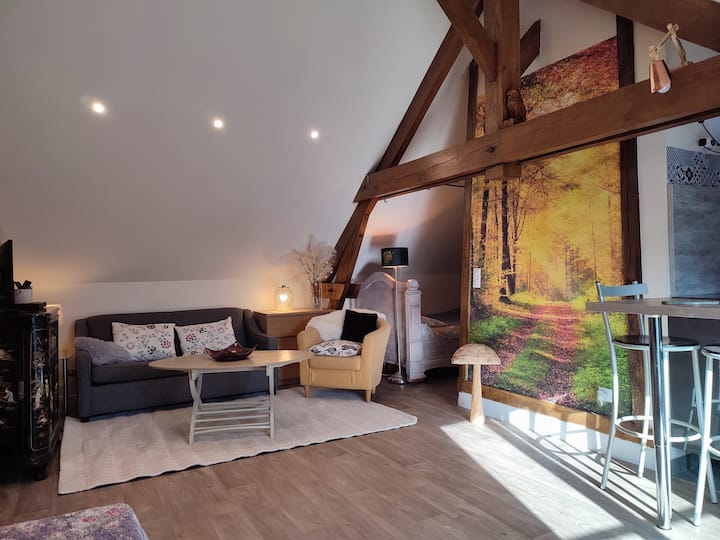This photograph captures the interior of a house that might be a studio apartment, showcasing a space thoughtfully divided into functional sections. The flooring throughout is light brown, resembling a laminate or hardwood finish, contributing to the cozy and warm atmosphere.

On the right side, there's a dining area with high stools featuring backs, positioned beside a small table. Behind this seating area, against the far right wall, there's a bed adorned with white floral bedding and an off-white headboard. The ceiling, painted white along with the walls, showcases exposed wooden beams and an A-frame structure, creating a rustic yet modern aesthetic.

The far wall hosts a blue couch adorned with throw pillows, adjacent to a beige chair. A beige rug lies underneath this seating arrangement, enhancing the cozy feel of the space. In front of the couch sits a table, likely for dining or lounging purposes. Additionally, a large piece of artwork depicting a trail in a forest hangs on one of the walls, adding a touch of nature to the room.

Several pieces of furniture, including a black dresser on the far left and a uniquely shaped mushroom lamp standing in front of the artwork, are strategically placed throughout the room. The sun streaming in creates a reflected shape of a window on the floor, illuminating the space and highlighting its welcoming ambiance.